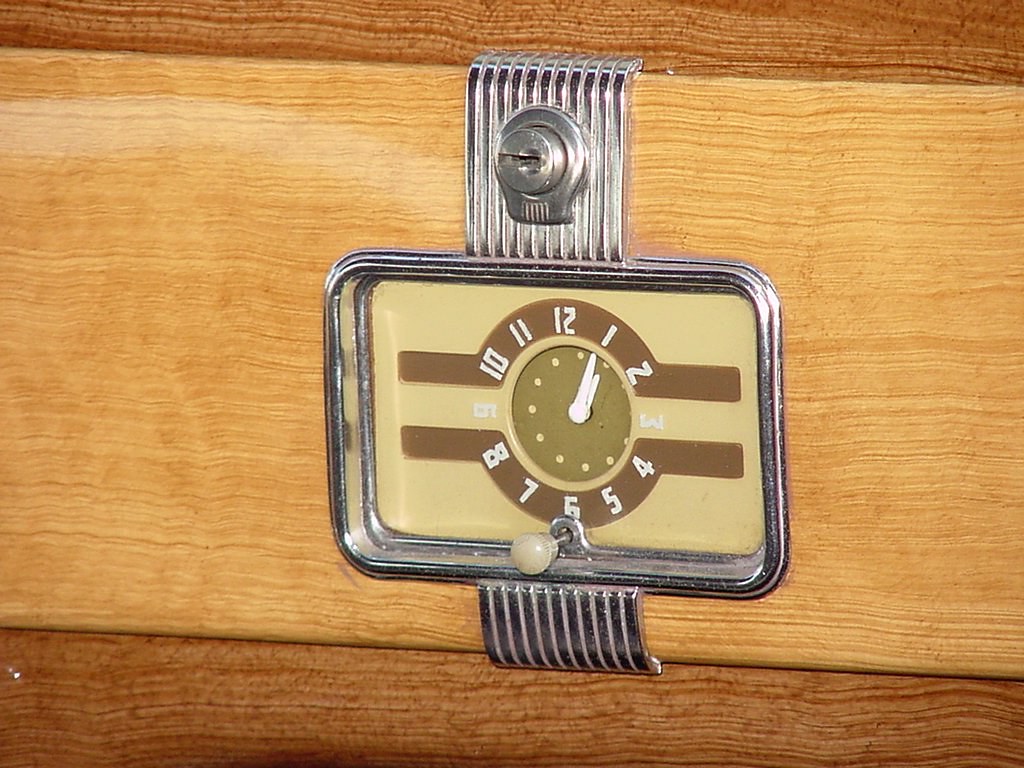A rectangular photograph showcases the intricate details of a vintage clock face. The centerpiece of the image is a square-shaped clock, elegantly encased in a silver frame. This frame is affixed to a large, light brown, natural wood surface, which itself is bordered by a dark brown base at the bottom and a dark brown top piece above. The face of the clock is protected by a transparent cover, possibly made of glass or plastic, revealing the light brown clock face adorned with dark brown lines both above and below it.

Adding a touch of old-world charm, a rectangular, ridged metal piece with a prominent key lock, turned to the side, is positioned above the clock frame. A similar ridged metal detail is found beneath the clock, contributing to its vintage aesthetic. The meticulous craftsmanship and the harmonious blend of colors and materials evoke a sense of timeless elegance, capturing the essence of an era gone by.